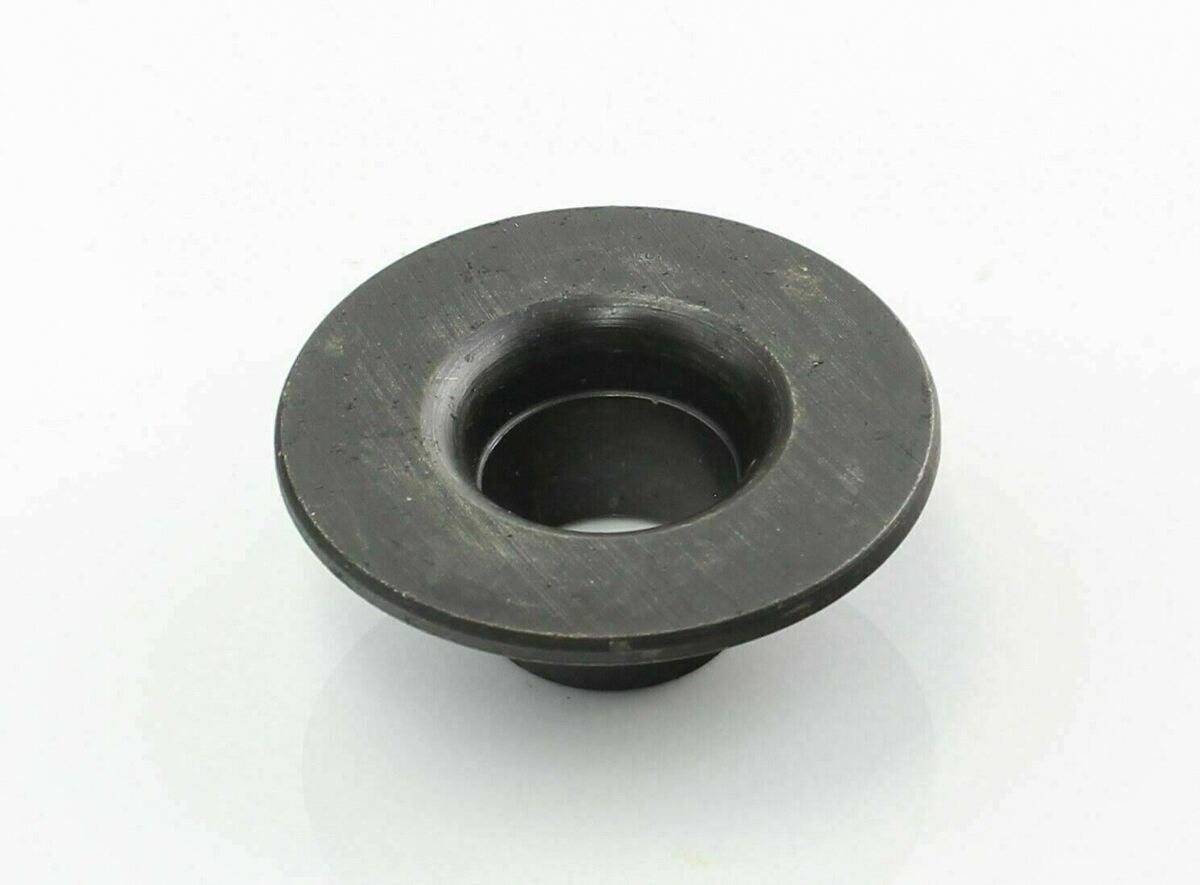The image depicts a black metallic component set against a white background. Centrally featured, the object resembles a composite washer with distinctive characteristics. Its upper part showcases a wider, flat circular surface that tapers into a smaller, deeper throat leading to a narrow round piece at the bottom. This design gives it an appearance akin to an inverted light bulb socket or a small metal bowl with its smaller opening facing the surface. The metallic item displays slight wear and accumulated sediments on its wider, more exposed surface, hinting at its practical use, possibly as a nut or a valve-like component. The clean white background accentuates the details and texture of the black metal piece.